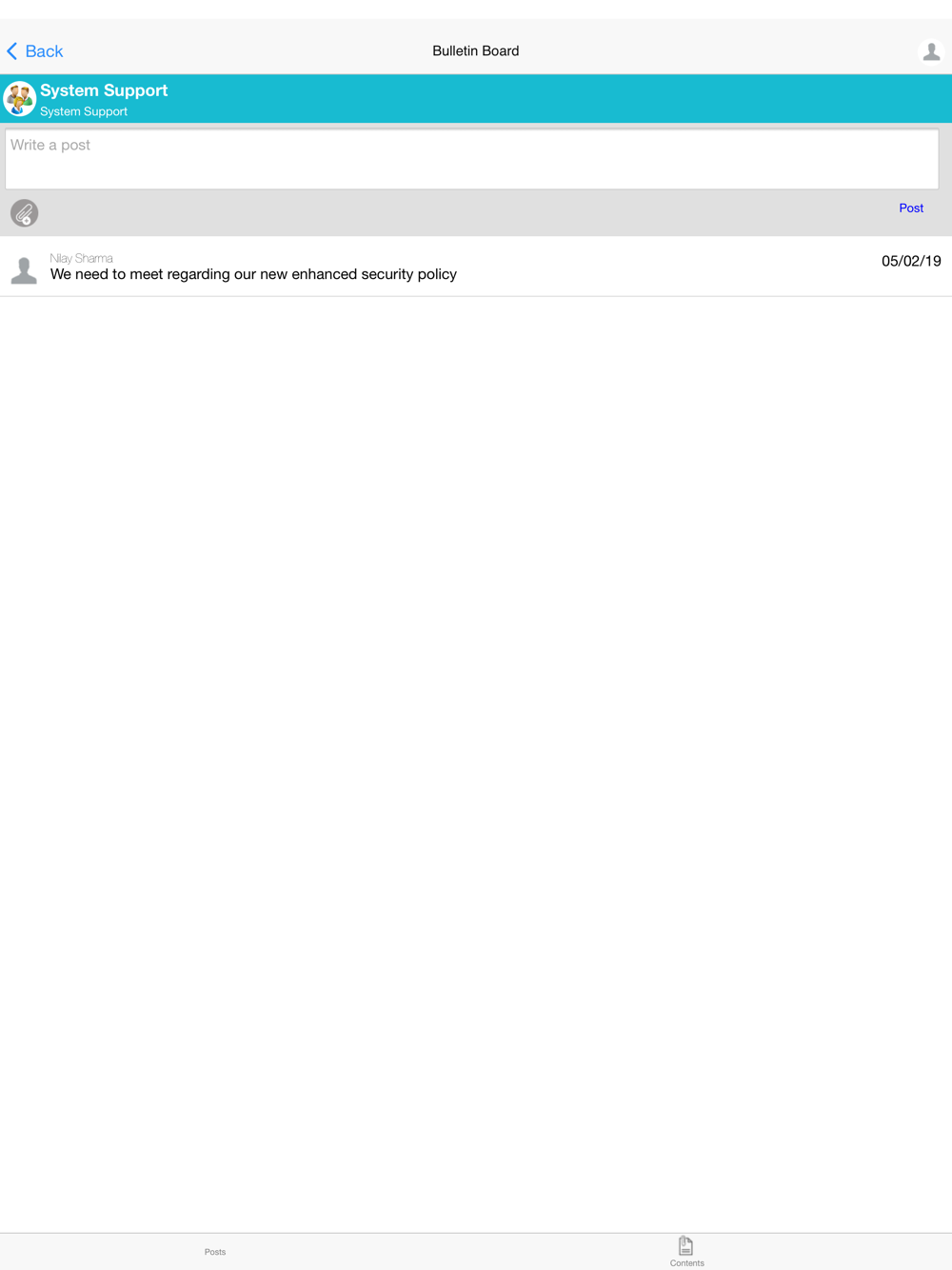The image features a user interface for a bulletin board system. The background at the top section is a very light gray, almost off-white color. On the left-hand side, there is the back end of a blue arrow followed by the word "Back" written in bold with a capital 'B'.

Towards the center, in a bold black font, the text reads "Bulletin Board," with both words capitalized. On the extreme right-hand side, there is an icon depicting the outline of a person, rendered in gray inside a white circle. 

Further down on the left side, there is another white circle containing three animated figures. Beside this circle, the text "System Support" is written in white, both words capitalized, and directly underneath, the same text appears again but not in bold.

The background transitions to a darker gray color below this point. In this gray section, there is a white rectangle followed by a row featuring a gray circle with a white paper clip icon inside it, and another white circle with a gray plus sign.

At the bottom right-hand corner, the word "Post" is displayed in blue with a capital 'P'. Directly under this word, in gray text on a white background, the name "Nyla Sharma" is presented. In bold black text below, it states, "We need to meet regarding our new enhanced security policy." This message was posted on 05/02/19.